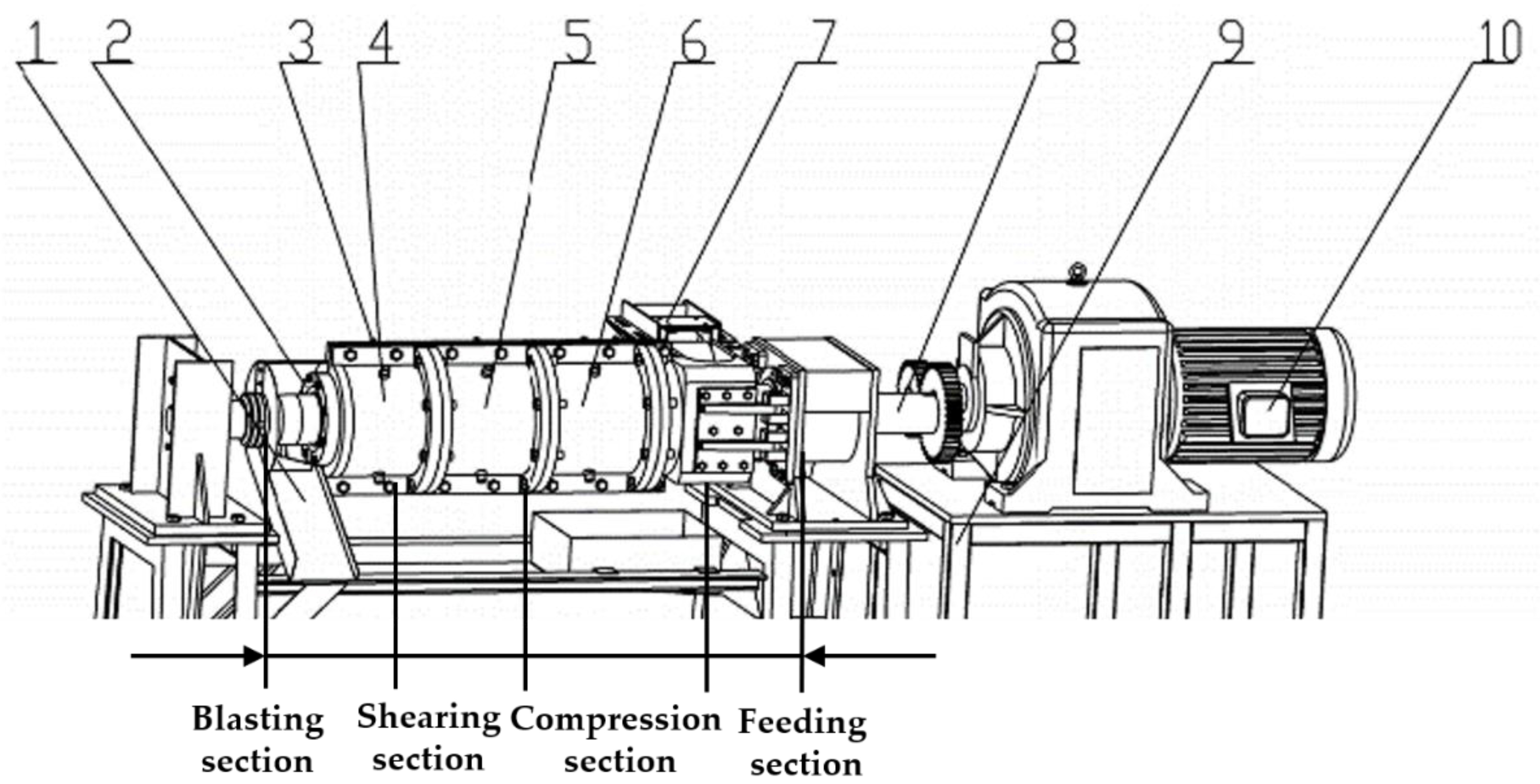The black-and-white hand-drawn image depicts a detailed diagram of a large, cylindrical machine, likely capable of rotating. The machine features several numbered labels from 1 to 10, each connected to different parts of the machine via black lines. At the bottom of the diagram, there are distinct sections labeled "blasting section," "shearing section," "compression section," and "feeding section," which are part of a long tube located towards the left side of the machine. The diagram also includes black arrows with triangular tips pointing to various components, adding to the detailed nature of the illustration. The machine appears to have a motor at the back and visible gears throughout, suggesting it might function by spinning and processing materials through these sections. Additionally, a black-colored handle is visible, which could indicate a manual or mechanical operation element. Despite the detailed depiction, the exact function of the machine remains unclear due to the stylized, minimalist nature of the drawing.